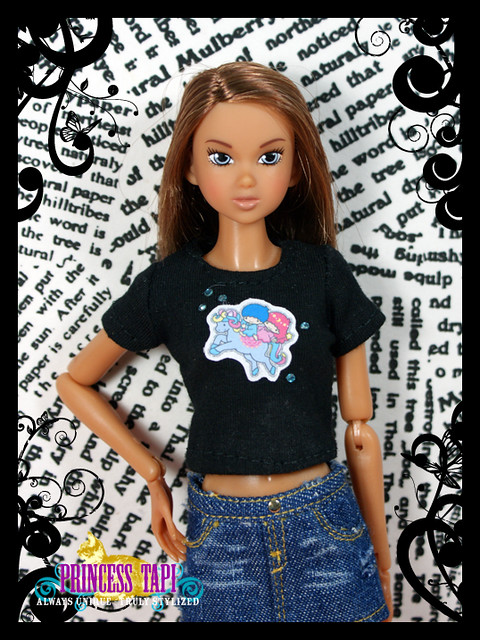This vibrant image captures a teenage Barbie doll figure as its focal point. With long brown hair and piercing blue eyes, the doll exudes a youthful, model-like essence. She is dressed in a stylish black shirt featuring a logo with two cartoon characters riding an animal—one with blue hair and one with pink or red hair—adding a whimsical touch to her outfit. Complementing her top is a trendy jean skirt. Positioned centrally, the doll's right arm is bent at a 90-degree angle, hand resting on her hip, while her left arm hangs naturally by her side. The backdrop is a creative collage of newspaper clippings arranged in various directions, adding an eclectic feel to the scene. The bottom left corner of the image is adorned with pink letters spelling out "Princess Tepi," followed by the phrase "Always un-mute, truly styled" in white letters. A black border embellished with butterfly designs frames the entire image, enhancing its artistic appeal.